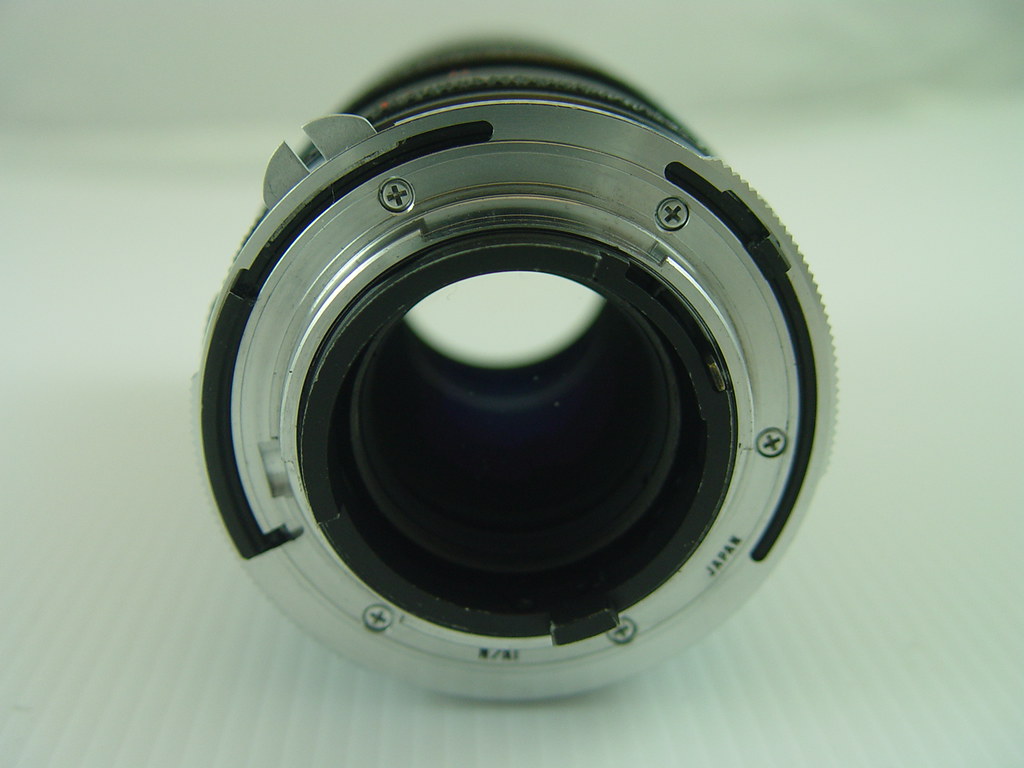This is an image of a camera lens or a similar cylindrical connection device, potentially the back of a camera lens that connects to the camera body. The device is primarily made of stainless steel with notable black areas, some of which might be hard plastic or metal. It features a black circular section in the center, surrounded by five screws. At the top left and bottom right, there are small metal teeth or stoppers designed for secure attachment. The background is white and slightly blurred towards the top and bottom, providing contrast to the detailed texture of the device, including the ridges and the engraved label 'Japan.' The lens appears to have depth, indicating potential for an extended or internal black component.